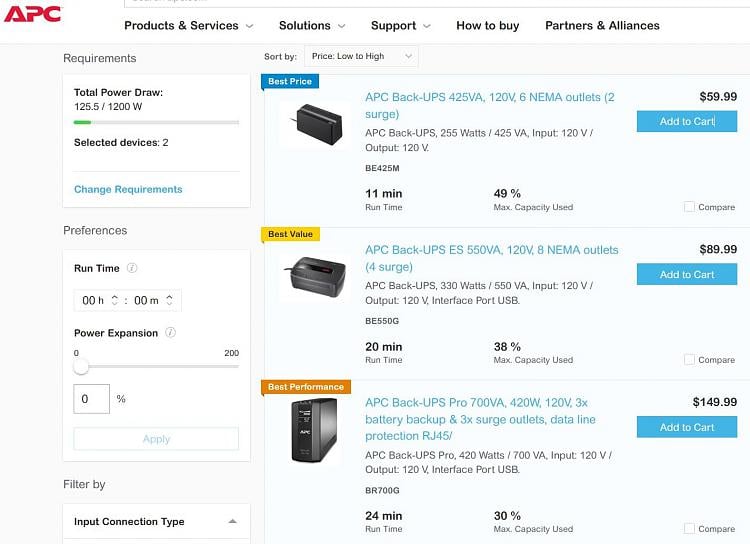In the image, the top left corner prominently displays the logo "APC" in blocky red lettering. The design is distinctive: the tail of the 'A' is positioned at the bottom, and the 'P' has a missing section towards the left.

On the right side, there's a navigational menu featuring black font text. The menu includes options such as "Products and Services," "Solutions and Support," each accompanied by arrowheads for dropdown menus. Further along, the options "How to Buy" and "Partners and Alliances" are shown without dropdown indicators.

The background transitions to light gray, with a white square area situated towards the upper left. Here, in bold black lettering, it reads "Total Power Draw:" followed by "125.5 / 1200 W" in non-bold text. A green progress bar indicates the power draw visually, with about one-tenth of the line filled in. Below this, another bold black label reads "Selected Devices:" followed by the number "2" in non-bold. A blue clickable link labeled "Change Requirements" is beneath yet another line divider.

Moving to the right, various products are listed, sorted by price from low to high. This filter is specified in a dropdown menu that reads "Price: Low to High." The first product, an "APC Back-UPS 14125 VA, 120V, 6 NEMA outlets (2 surge)" is priced at $59.99. Notably, the top left corner of the product listing features a yellow tag with the text "Best Value" in black.